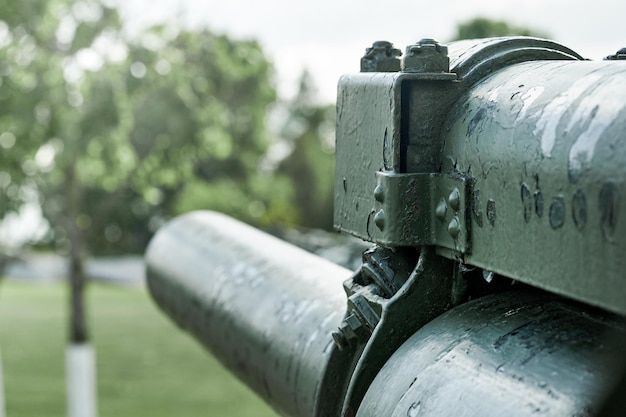The photograph captures a close-up view of a partially visible, army green artillery cannon in an outdoor park setting. The object is distinguished by its hefty steel structure, prominently featuring large bolts and rivets. The green paint on the metal shows signs of aging, with patches of flaking and rust visible. Cylindrical tubes protrude forward, indicative of artillery or missile launchers. While the artillery structure is in sharp focus, the background landscape with blurred trees and a grassy lawn provides a contrasting, out-of-focus backdrop, emphasizing the military equipment in the foreground.